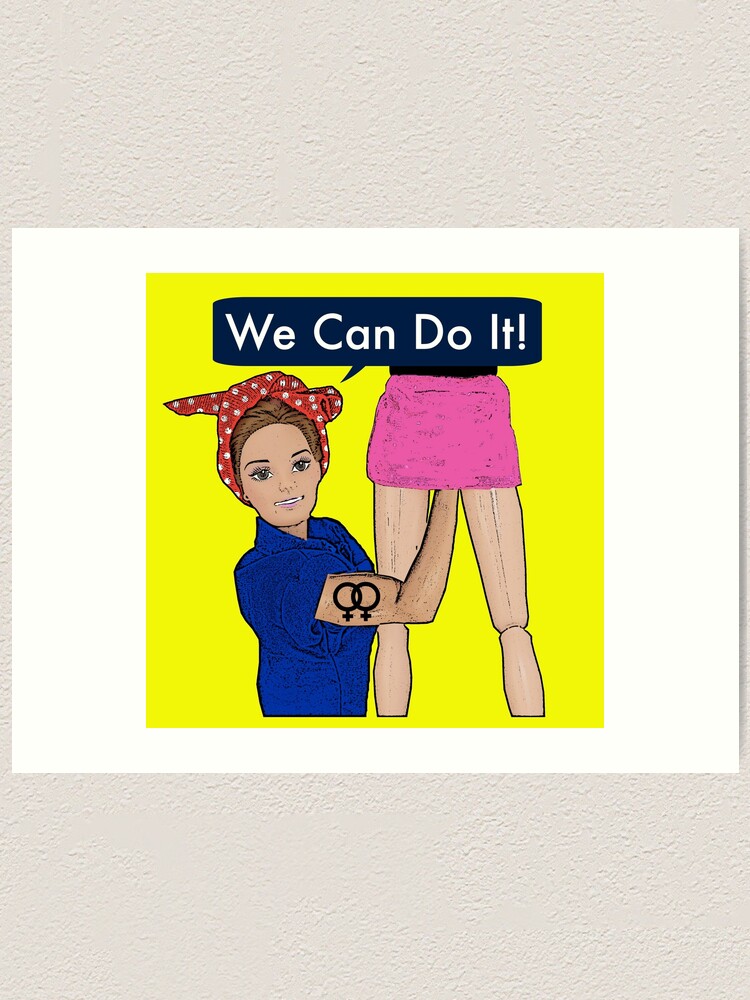The image in question is an illustration that appears to be inspired by Rosie the Riveter, depicted in a Barbie-like, animated style. Central to the composition is a woman with a red bandana tied over her brown hair, resembling the iconic Rosie the Riveter. This character with a flexed right arm shows two female gender symbols tattooed on her bicep and wears a blue shirt. A speech bubble next to her, rendered in blue with white text, emphatically declares "We can do it." The background of the illustration is a bold yellow square, framed by a white border which gives the appearance of the scene being part of a card or poster. Below Rosie's flexed arm, she is seen reaching upwards beneath the hem of another female figure's short pink miniskirt. This second figure is only partially visible, showing just her legs and miniskirt. The two characters have the segmented, articulated limbs reminiscent of dolls, further enhancing the Barbie-like aesthetic. The overall imagery combines feminist iconography with a playful yet provocative twist.